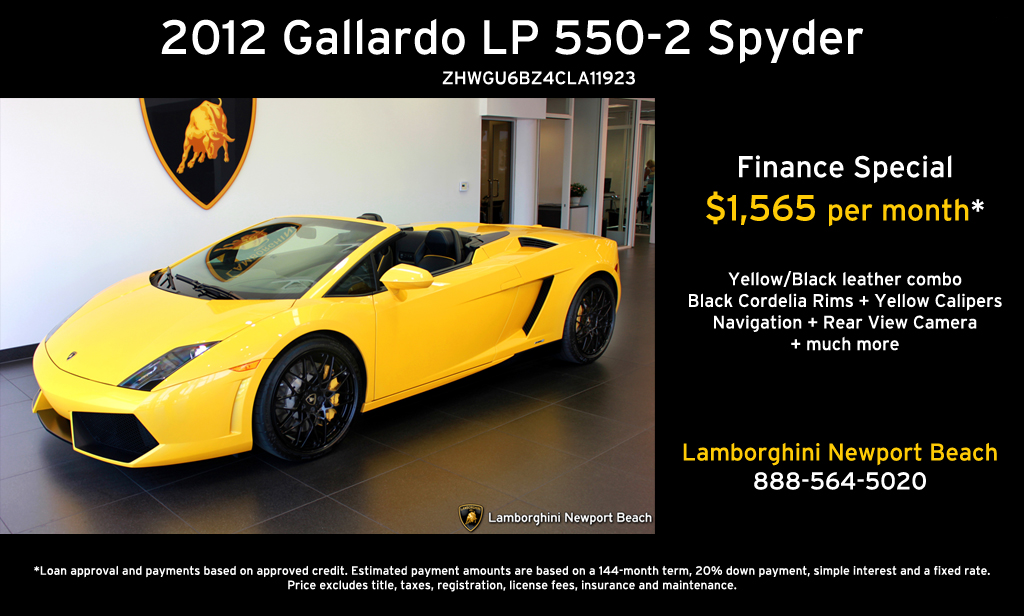This advertisement for the 2012 Gallardo LP 550-2 Spyder, prominently displayed against an all-black background, showcases a striking yellow and black convertible sports car. The top section of the ad features the car model name "2012 Gallardo LP 550-2 Spyder" in white letters, followed by a vehicle identification number. Beneath this, a vibrant image of the car is positioned on the left, revealing its sleek, low-profile design, black Cordelia rims, and yellow calipers, indicative of its high-performance capabilities. The car, shown in a showroom setting, highlights its black leather interior and distinctive yellow exterior. To the right of the image, the ad promotes a Finance Special, detailing a $1,565 per month rate in bold yellow text. Additional information includes details like black leather combo seats, enhancing the luxurious appeal of the vehicle. The ad concludes with the dealership name, Lamborghini Newport Beach, and provides their contact information, all formatted in a cohesive theme that mirrors the car's yellow and black color scheme.